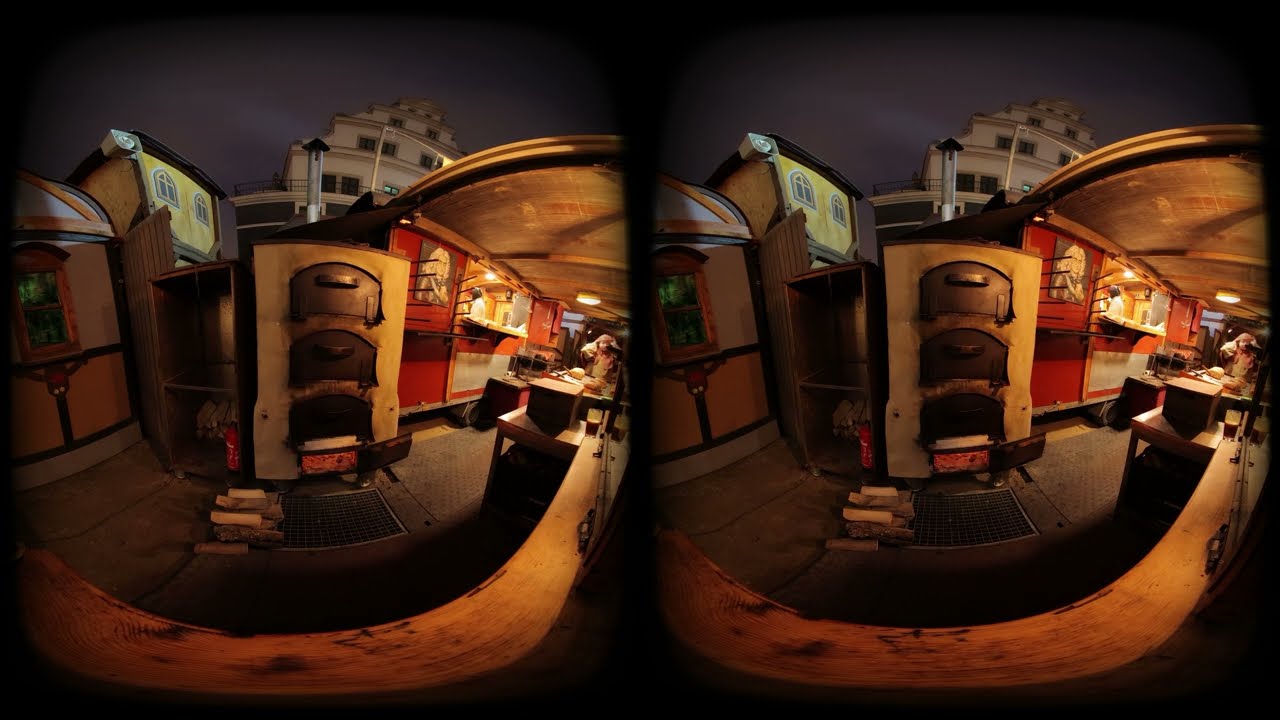The landscape-oriented image features two identical, side-by-side, square-shaped, fisheye distorted snapshots of the same outdoor night scene, giving a 360-degree effect. The scene is set against a dark gray night sky, with a backdrop that includes a three or four-story building and a tan or yellow-walled structure with white-framed windows and a dark roof. In the foreground, under a white metal awning, there appears to be a cabinet or stack of three metal drawers or chutes, potentially functioning as a kiln or fireplace, with metal grates and chopped firewood nearby. Additional whimsical elements and possibly a two-story shelf are present, but their details are skewed by the fisheye effect, rendering them less discernible. Decorative portraits and objects line an orange wall within this eclectic mix, enhancing the scene's enigmatic and historical ambiance.